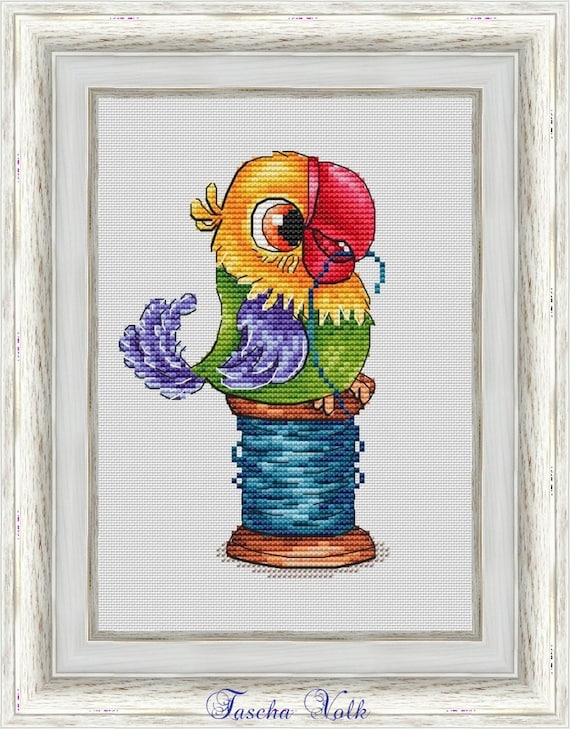The image showcases a detailed cross stitch picture framed in a light white wooden frame with an off-white or plastic inlay. At the bottom of the frame, written in cursive and a flowery script, is the name "Tasha Volk". The focal point of the stitched artwork depicts a multicolored parrot perched on a brown wooden spool of light blue thread. The parrot's body is green with purple wings and a purple and white tail, while its head is yellow gold with striking orange eyes and a bold, bright red beak grasping some blue thread. The composition is set against a white background, bordered by a slightly darker shade, possibly a light grayish brown, within the frame, giving the whole image a neatly contained and clean look. The photograph has a vertical orientation, emphasizing the elegant and vibrant details of the parrot and the spool of thread.